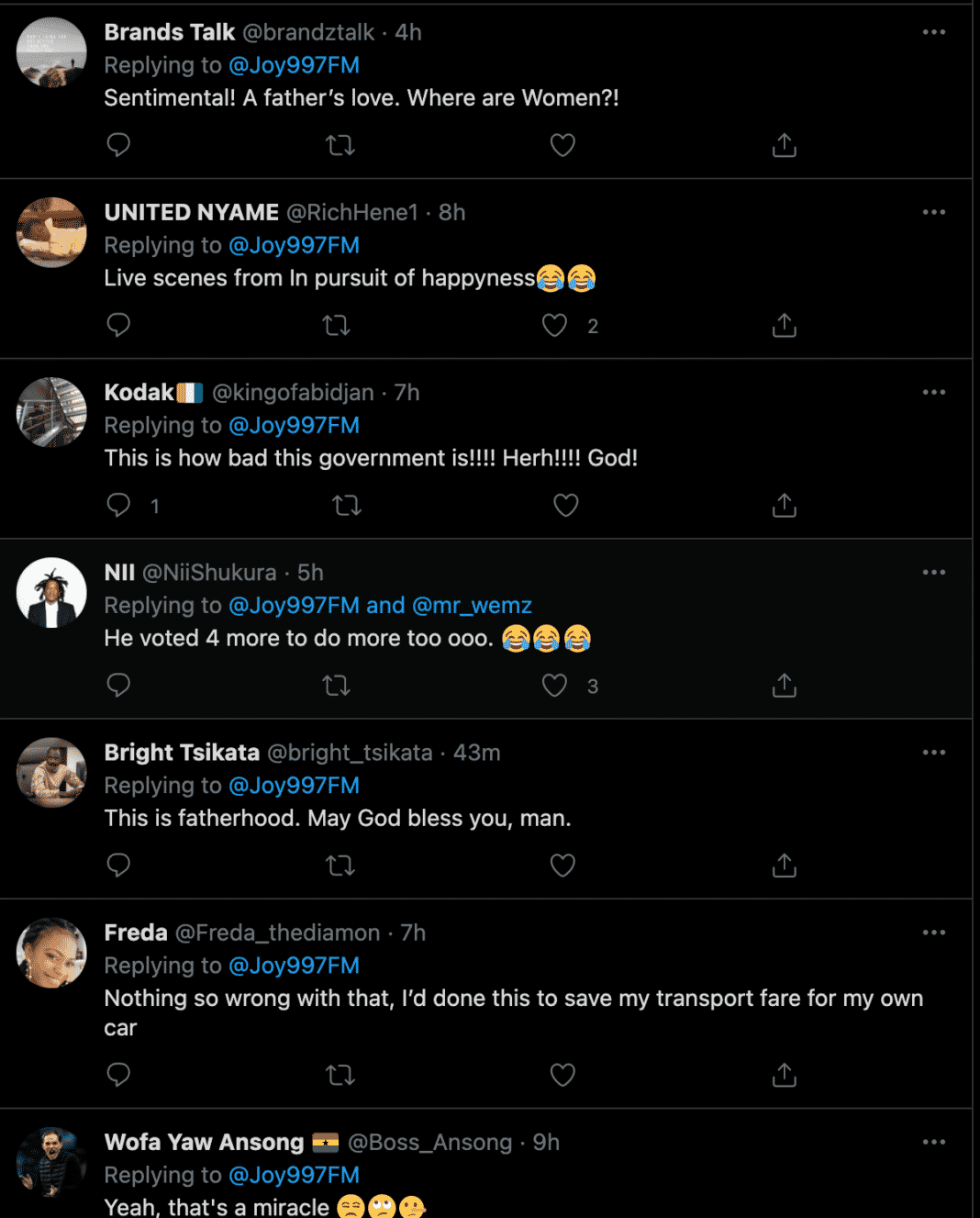The image depicts a Twitter post with a black background featuring a thread of comments from various users. The primary tweet, posted by @BrandsTalk, reads "Sentimental at Father's Love. Where are women?" and was posted four hours ago. Below this tweet, @UnitedNYAE replied eight hours ago with the comment, "License from In Pursuit of Happiness," accompanied by two laughing-crying emojis. 

Next, a user named Kodak (@KingOfAbidjan) responded seven hours ago, commenting, "This is How Bad This Government Is, HERH!!! God!!!" showing clear frustration. Further down, user Nii (@Nyshakur) replied five hours ago, saying, "Replying to @Joy997FM and @Mr_WEMZ, he voted for more to do more to," followed by three laughing-crying emojis, indicating a humorous take. 

Another user then chimed in with the comment, "This is Fatherhood, may God bless you, man," suggesting support and admiration. Finally, a different user adds, "Nothing's so wrong with that, I done this to save my transport fare for my own car," sharing a personal anecdote in the context of the discussion.

The thread exemplifies a diverse range of reactions, from humor and frustration to support and personal stories, centered around the original tweet on sentimental aspects of fatherhood.